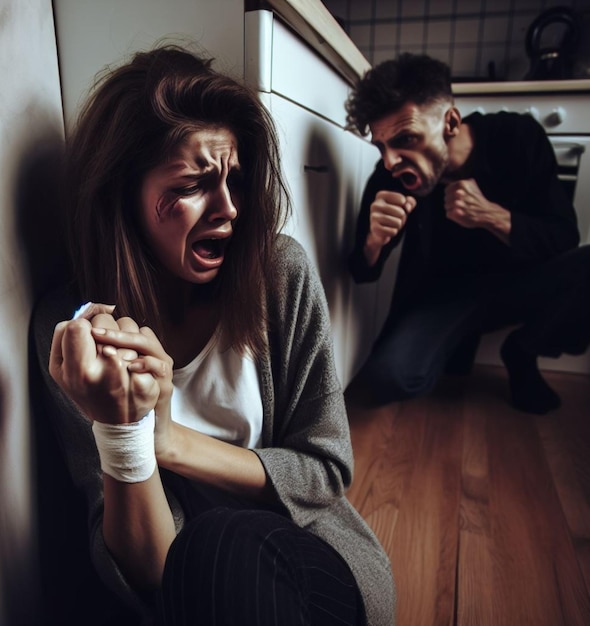In this unsettling image, set in a modern kitchen with white countertops and a stove in the background, a woman is depicted sitting on the floor to the left. She is crouched and appears deeply distressed, with a cut near her right eye and a bandage around her right wrist. Dressed in a gray sweater, white shirt, and dark pants, she is clasping her hands together, possibly crying out in fear or anguish. Her expression is one of palpable terror, directed toward a menacing man in the right corner. This man, with dark curly hair, is dressed entirely in dark clothes and has an aggressive, clenched-fist stance. His facial expression is equally frightening and filled with rage. The scene is further accentuated by the hardwood flooring and wooden-grained tile, enhancing the overall sense of dread. The photograph, which may be computer-generated, vividly portrays an alarming moment of intimidation and emotional distress.